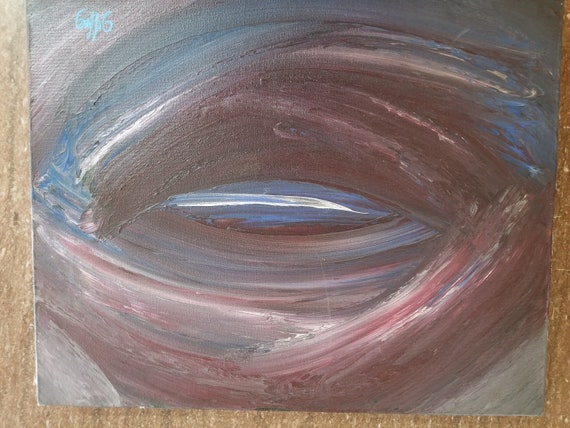The image depicts an abstract oil painting on a canvas wall art set, placed on a brown or potentially stone surface, illuminated by natural light coming from the top left, creating a slight glare. The painting, in a landscape orientation, lacks frames and features heavy, layered brush strokes forming an intricate, eye-shaped pattern without a pupil. The swirling, almost counterclockwise movement of the brush strokes creates a fluid pattern that evokes the inside of a wave. The color palette is a complex blend of grays, silvery gray around the edges, blue-gray, and rich wine, maroon, silver, and pink shades, with a blue center highlighted by a white line. This eye-like shape is surrounded predominantly by gray hues, interspersed with touches of white. The top left corner of the canvas bears the artist's signature in light blue, with characters that appear to begin and end with the letter 'G,' though they are not entirely legible.